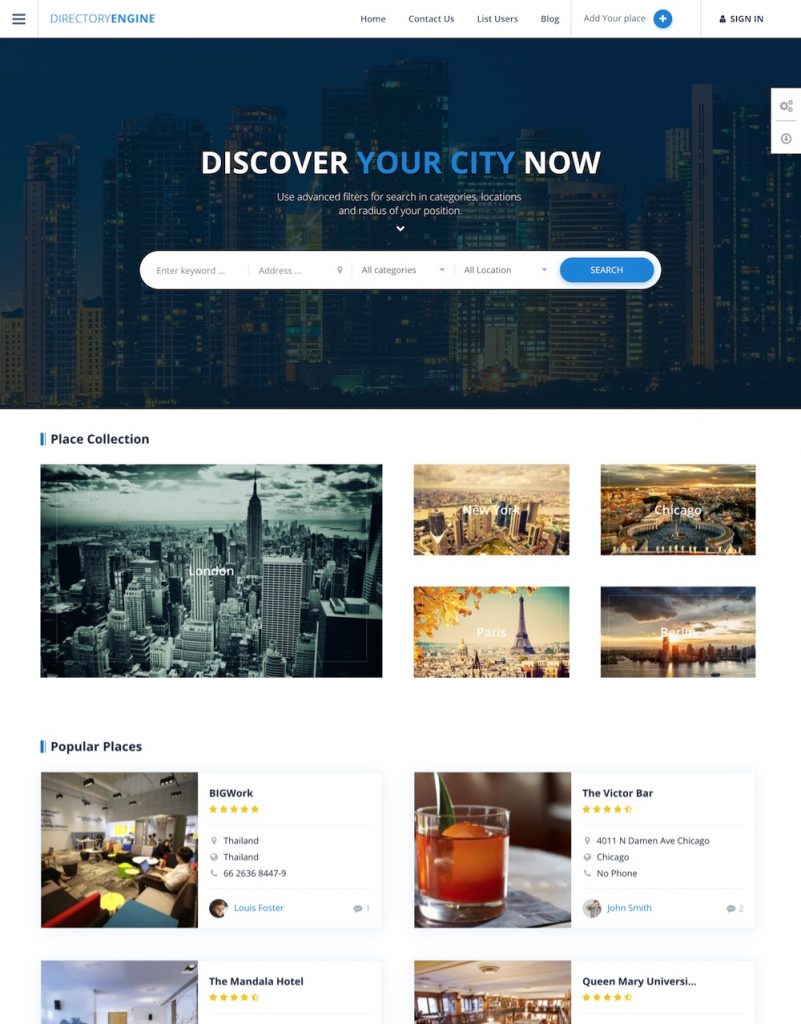This screenshot captures a web interface of a site named "Directory Engine". At the top of the page, a navigation bar offers various clickable options such as "Home," "Contact Us," "List Users," "Blog," and "Add Your Place." A notable element is a blue circle with a white plus sign, indicative of additional options. Positioned at the far right of the navigation bar is the 'Sign In' option, accompanied by a silhouette of a person.

Dominating the center of the screen is an image depicting a cityscape at dusk, with several buildings illuminated against a darkening sky. The photo has a muted tone, ensuring the text overlay remains prominent. Across the upper section of the image, the slogan "Discover Your City Now" is prominently displayed, with "Discover" and "Now" in white and "Your City" in blue, drawing visual emphasis.

Beneath the slogan, there is a comprehensive search bar inviting users to "Enter a Keyword, Address, All Categories, All Location," with a large search button to initiate the query. An advisory tip above the search bar suggests users to "Use advanced filters for search in categories, locations, and radius of your position" for more refined results.

Further down the page, the site offers two distinct sections to explore: "Place Collection" and "Popular Places," each containing clickable images and descriptions for more information and navigation. The overall design clearly aims to facilitate a user’s exploration and discovery of city-specific information effortlessly.